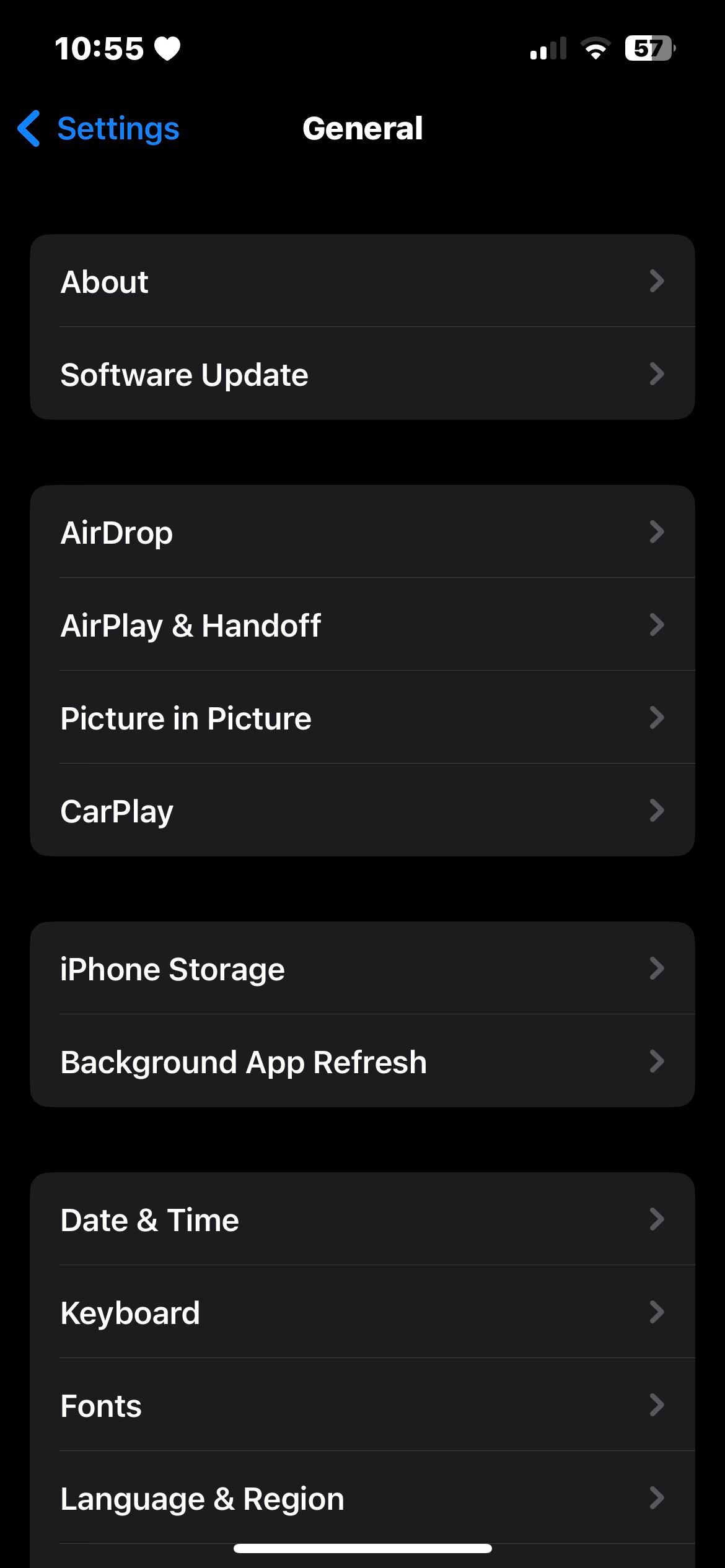The image depicts a smartphone screen set against an all-black background. At the top of the screen, white text and icons are displayed. In the upper-left corner, the number "10:55" is shown, accompanied by a white heart icon to its right. On the upper-right side, indicators for connectivity and battery life are visible: two out of four Wi-Fi bars, a Wi-Fi signal icon, and a battery icon showing 57%.

Below this top section, centrally positioned in bold white text, is the word "General." To the left of "General," there is a blue left-facing arrow and the word "Settings" in blue.

The main portion of the screen is divided into several lines, each featuring a bold white label with a corresponding gray forward arrow on the right-hand side. The lines read as follows:

1. **About**
2. **Software Update**
3. **AirDrop**
4. **AirPlay & Handoff**
5. **Picture-in-Picture**
6. **CarPlay**
7. **iPhone Storage**
8. **Background App Refresh**

Following a small black divider, the next section, also in bold white text, includes:

1. **Date & Time**
2. **Keyboard**
3. **Fonts**
4. **Language & Region**

At the very bottom edge of the screen, there is a wide horizontal white line, completing the minimalist and monochromatic design of the interface.